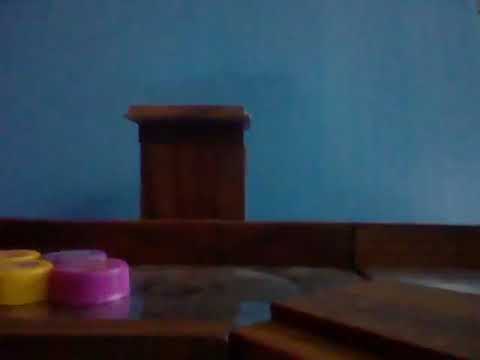The image showcases a brown wooden desk with some obvious imperfections, such as dust and smudges that obscure its glossy surface. On the bottom left corner of the desk, there are four clustered plastic bottle caps: two yellow ones on the far left, one pink cap prominently in the foreground, and a purple cap in the background on the right. The desk also features a secondary platform on the bottom right, adding a layered effect to its structure. A dark wooden lip runs along the back edge of the desk, leading to a blue wall with a brown doorway featuring wooden trim in the backdrop. The overall image suffers from significant compression artifacts, making it difficult to see details clearly.